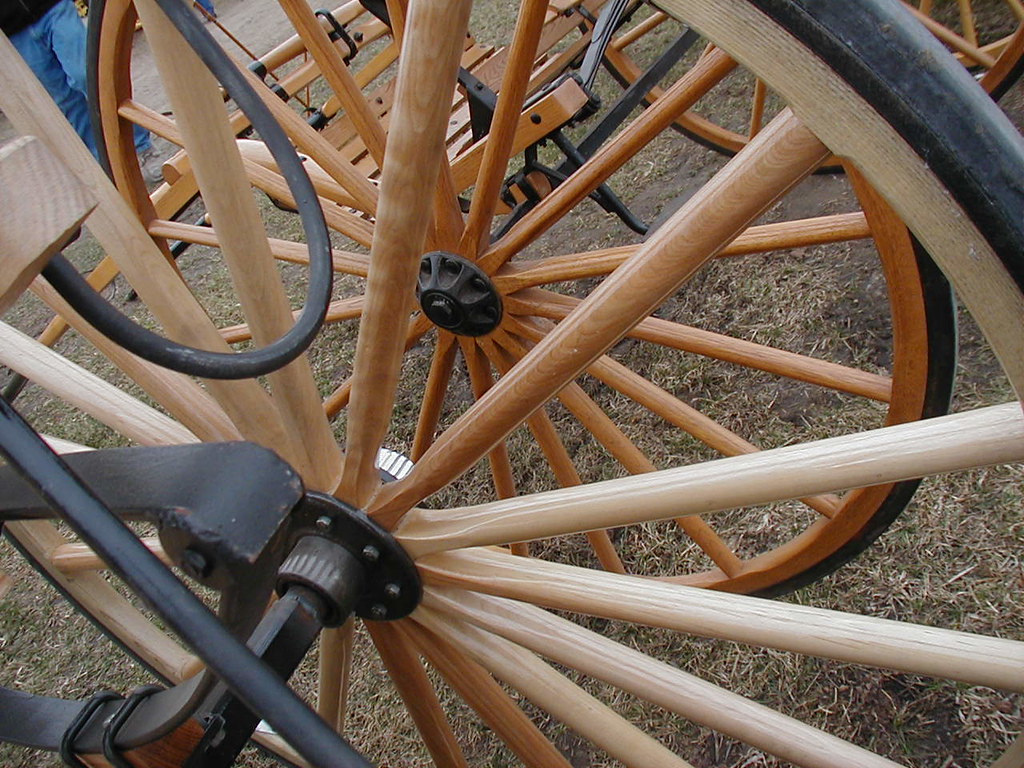The photograph showcases a detailed, close-up view of two wooden wagon wheels situated in a dirt field with sparse, dried grass. The foreground wheel features polished, light-colored wooden spokes and a wooden frame, possibly coated with a layer of rubber or metal. This wheel is connected by a black metal axle with additional metal components visible. Just behind this, the second wheel, made of a slightly darker wood, mirrors the first in materials and construction, both with a dark metal piece at the center securing the wheel to the axle.

Further details reveal straps and black metal hardware reinforcing the wheels and their connection to the wagon. In the background, a wooden bench or possibly a small chair can be observed, also secured with black metal fixtures. The scene is complemented by the presence of a person wearing blue jeans and a black top, walking past the carts. Another set of blue jeans and footwear is also faintly visible, indicating another person nearby. The field setting appears dormant for winter, with patches of muddy and brown grass scattered about.